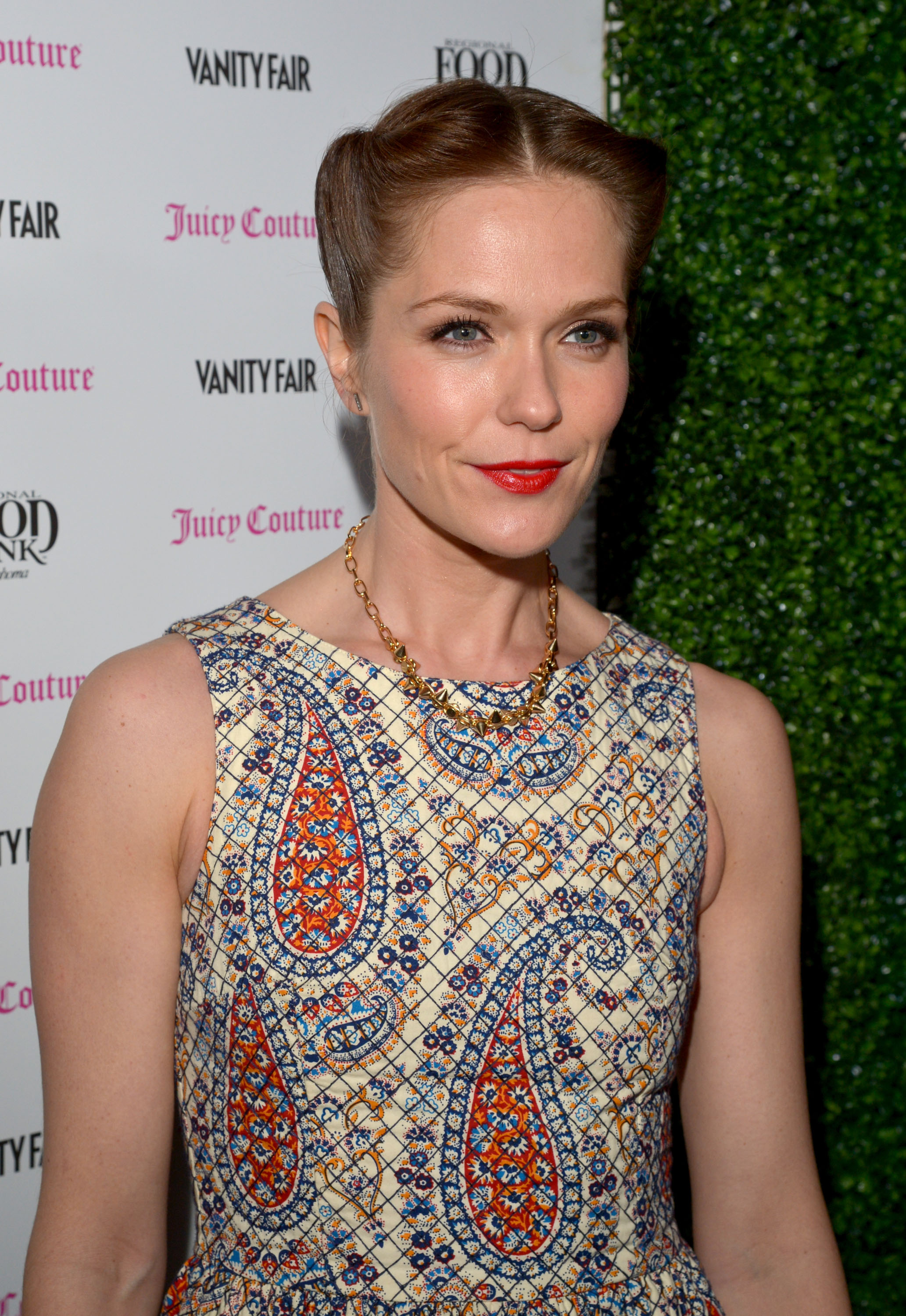The image captures a famous woman, possibly a model or actress, standing and smiling brightly with striking red lipstick. Her hair is elegantly pulled up into a bun, revealing a clear and radiant face. She is wearing a sleeveless, crop-style top adorned with intricate paisley patterns in hues of orange, blue, and white. Around her neck, she sports a gold chain-link necklace. To her left, a lush, high green hedge extends upwards, adding to the picturesque background. Behind her right shoulder, a white backdrop showcases the names "Juicy Couture" in pink font and "Vanity Fair" in black font, repeated in a patterned manner, suggesting a promotional banner likely from a high-profile event, perhaps a red carpet or award show.